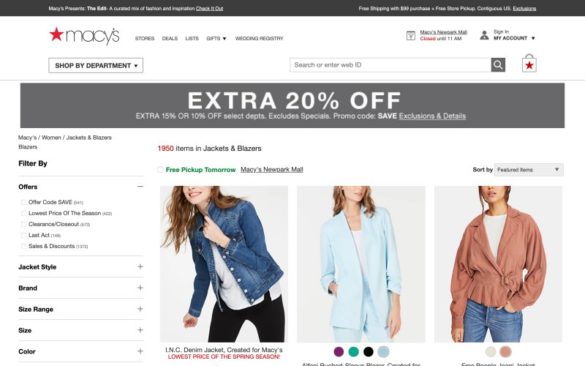This image captures a detailed view of a Macy's shopping webpage. Prominently displayed at the top is the Macy's logo, followed by sections labeled "Stores," "Deals," "Gifts," and "Wedding Registry." The search box, which invites users to "search or enter web ID," is situated near these sections. 

Highlighted across the top banner is a promotional message detailing an "extra 20% off," as well as "extra 15% or 10% off select departments," while specifying exclusions, specials, and the necessary promo code “SAVE.” It also links to further exclusions and deals.

Central to the page are three images depicting fashionistas modeling different stylish dresses. To the left side of the page, a navigation menu allows users to filter products by categories such as offers, jacket style, brand, and size. The comprehensive layout aims to provide a seamless shopping experience, integrating visually appealing content with practical navigation options.